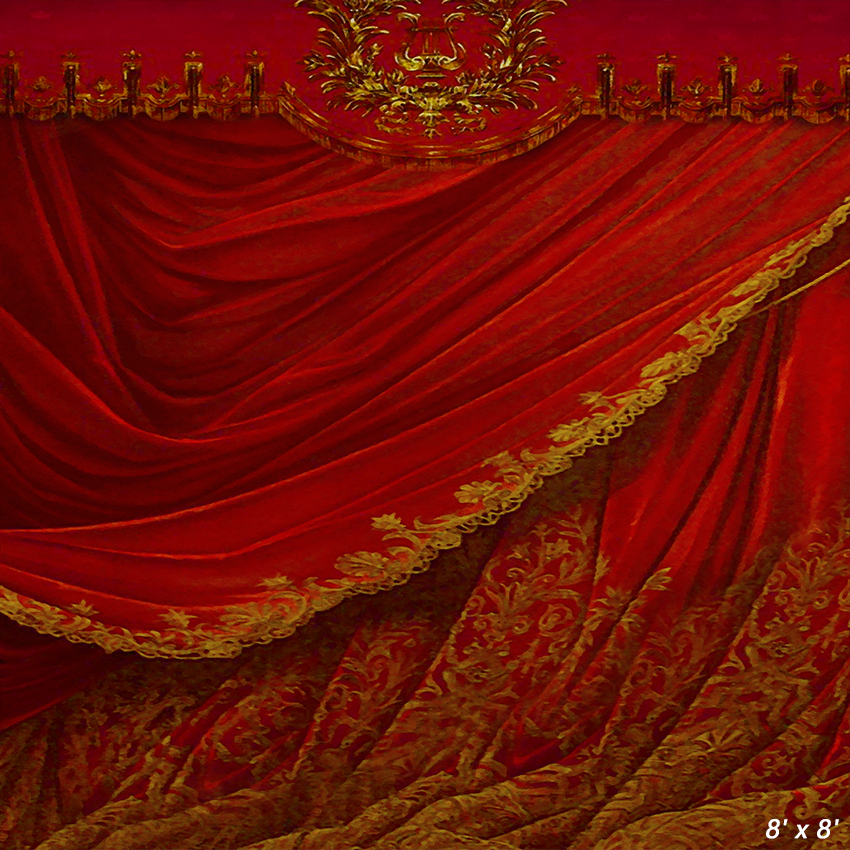This image captures a lavish, voluminous red curtain with an ornate, royal appearance. The curtain is adorned with intricate gold trim and boasts a brocaded design with detailed patterns. At the top, there is a regal insignia or crest consisting of gold and yellow floral and leaf motifs. The curtain's rich folds and gathered fabric suggest it belongs to an old theater or a grand European palace. In the bottom right corner of the image, there is white text indicating the dimensions, "8 feet by 8 feet."